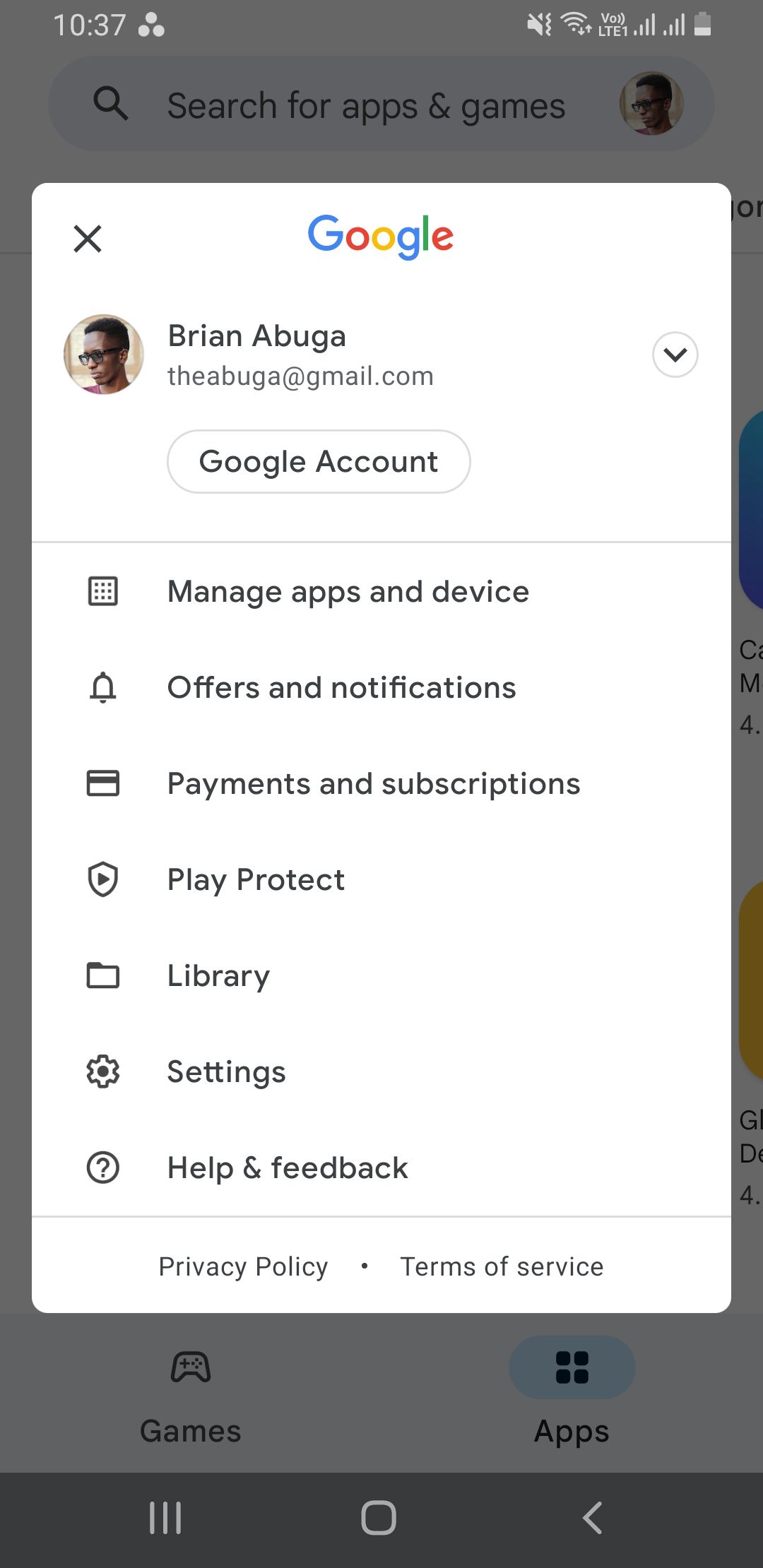This screenshot captures a mobile interface of a Google account settings page, prominently featuring the user profile of Brian Abuga, whose email is theabuga@gmail.com. The interface is part of a pop-up window, evident from the grayed-out background, indicating that Brian accessed this page while visiting a different section of a Google website, possibly for configuring his account or managing his settings.

The pop-up window highlights several key options available for managing various aspects of his Google account. These options include:

- **Manage apps and device**
- **Offers and notifications**
- **Payments and subscriptions**
- **Play Protect**
- **Library**
- **Settings**
- **Help and feedback**

At the bottom of the pop-up, links to the **Privacy Policy** and **Terms of Service** are provided for additional reference.

The screenshot also shows typical mobile interface elements, such as the status bar at the top with the battery percentage, current time, and data signal indicators. Below the main content area, standard navigation buttons for mobile devices, including tabs and a back button, are visible.

In the background, faint outlines of other content such as games and apps suggest this pop-up appeared over another section of the website. This detailed capture provides a comprehensive view of the options available in the Google account settings on a mobile device.